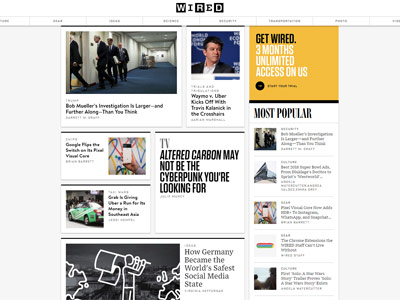Screenshot of a Wired Magazine Website

This colorful screenshot captures the homepage of the renowned technology media website, Wired. At the top of the page, the distinctive Wired logo is prominently displayed, featuring a black, white, black, white letter pattern. The site showcases a variety of articles beneath the logo, each reflecting Wired's focus on tech-related topics.

The articles presented include:

1. "Bob Mueller's Investigation is Larger and Further Along Than You Think" – This piece, recalling events from several years ago during Trump's presidency, discusses the scope of Robert Mueller's investigation into Trump, which ultimately yielded no substantial outcomes.
 
2. "Waymo vs. Uber Kicks Off with Travis Kalanick in the Crosshairs" – This article appears to delve into the legal battles between the autonomous vehicle companies Waymo and Uber, highlighting former Uber CEO Travis Kalanick's involvement.

3. "Altered Carbon May Not Be the Cyberpunk You're Looking For" – A review or critique about the popular science fiction series "Altered Carbon," suggesting it may not meet certain cyberpunk expectations.

4. "Google Flips the Switch on Its [Unreadable] Core" – This article title is partially obscured but likely addresses a major update or change to one of Google's core technologies.

5. "How Germany Became the World's Safest Social Media State" – This article likely explores Germany's approach to regulating social media, possibly highlighting its safety measures and policies.

To the right side of the page, there is an advertisement offering three months of unlimited access to Wired's content, encouraging readers to subscribe and get "wired."